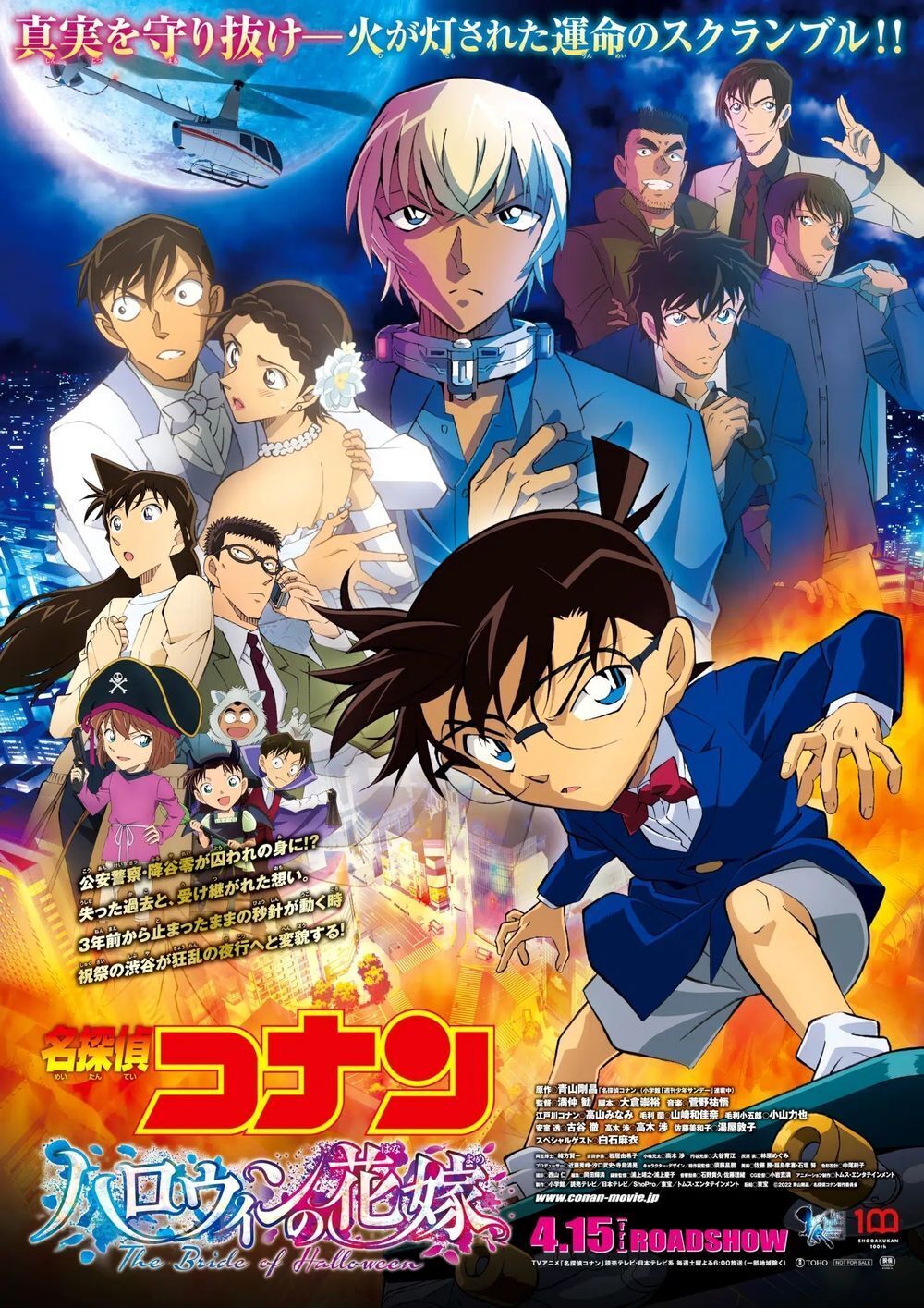The poster, rectangular and taller than it is wide, is an advertisement for an anime show. The poster is densely covered with Japanese anime characters and features Japanese writing at both the top and bottom. The only English text reads "The Bride of Halloween 4.15 Roadshow" in the bottom right corner. The central characters include a young boy in a blue suit and glasses, likely Detective Conan, among approximately 13 others. Key visuals include a helicopter flying against a moonlit night sky on the top left, with city lights in the background. A girl wearing a blue jacket and gray shorts with a bow tie is seen riding a green skateboard with yellow wheels. Additional characters portrayed in vivid detail include a girl in a pirate hat, a man in glasses talking on the phone, and a couple in wedding attire. A prominent feature is a fiery, yellow-orange border at the poster's bottom. The dynamic design of the poster highlights numerous animated figures and vibrant colors.